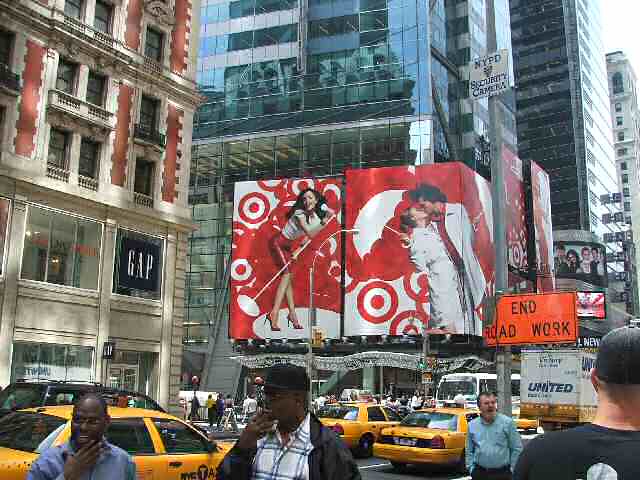The image was taken outdoors in what appears to be New York City, possibly near Times Square, during the daytime. It captures a bustling city street lined with tall buildings. Central to the image is a large building with mirrored glass windows, displaying red and white advertisements. One ad depicts a man and woman kissing under an umbrella, while the other showcases a woman singing into a microphone. To the left of this modern structure stands an older brick-and-stone building with a sign for GAP visible in one of its windows. 

Pedestrians crowd the sidewalks, with a diversity of people including a gentleman in a plaid shirt stroking his chin and another with sunglasses. Numerous yellow taxis and a white United moving van are prominently seen on the street, alongside a "End Road Work" sign. Notable figures include a man in a black t-shirt with a black baseball cap and another in a blue button-down shirt. Adding to the city's characteristic hustle, a NYPD security camera pole stands among the lively scenery. The image is slightly blurry, contributing to the sense of fast-paced urban life. The collective elements, from the architectural contrasts to the vibrant advertisements and busy street, vividly encapsulate the dynamic atmosphere of this iconic city location.